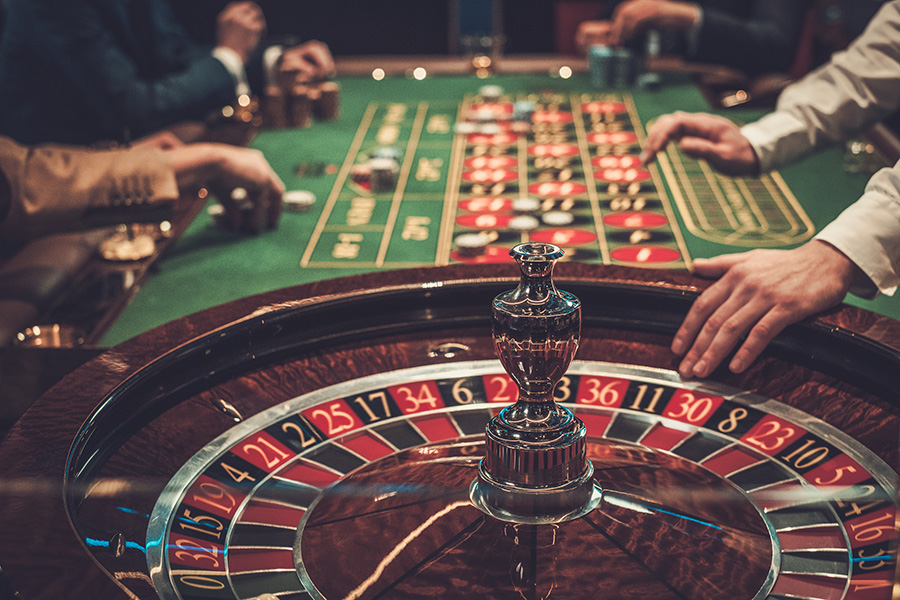The image depicts an indoor casino scene focused on a stationary roulette wheel at the forefront, held steady by the croupier's hands. Surrounding the wheel is a betting table populated by three seated gentlemen, each deeply engaged in the game. They have stacks of chips positioned in front of them, representing their bets on various numbers. One man has a significant amount of money placed on the sidebar, while the others have smaller bets dispersed across the table. The scene captures the anticipation and strategy inherent in gambling, as players await the outcome of the next spin.